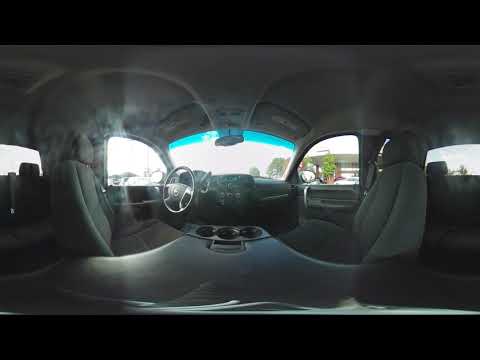The panoramic 360-degree photograph showcases the interior of a vehicle, most likely a car, with the evident distortions typical of such images. At the center of the image, the dashboard is prominently displayed, with a steering wheel positioned to the left. Both the driver's seat and the passenger seat are seen facing each other, exaggeratedly stretched due to the panoramic effect, with an abnormally wide divider separating them. Three distinct cup holders are situated in front of this divider. The entire scene is rendered in various shades of light and dark gray. The seats boast cloth upholstery, while the dash is fashioned from black plastic. Above, the windshield has a light turquoise tint at its top, enhancing the contrast of the natural daylight flooding the car's interior. The vehicle's roof is also visible, contributing to the comprehensive view of the car's interior layout. Both door panels and windows are clearly visible on either side, and the back of the vehicle is subtly included in the periphery of the image, featuring rear seat headrests and back windshield details. The absence of occupants further accentuates the spacious yet distorted ambiance of the car's interior.